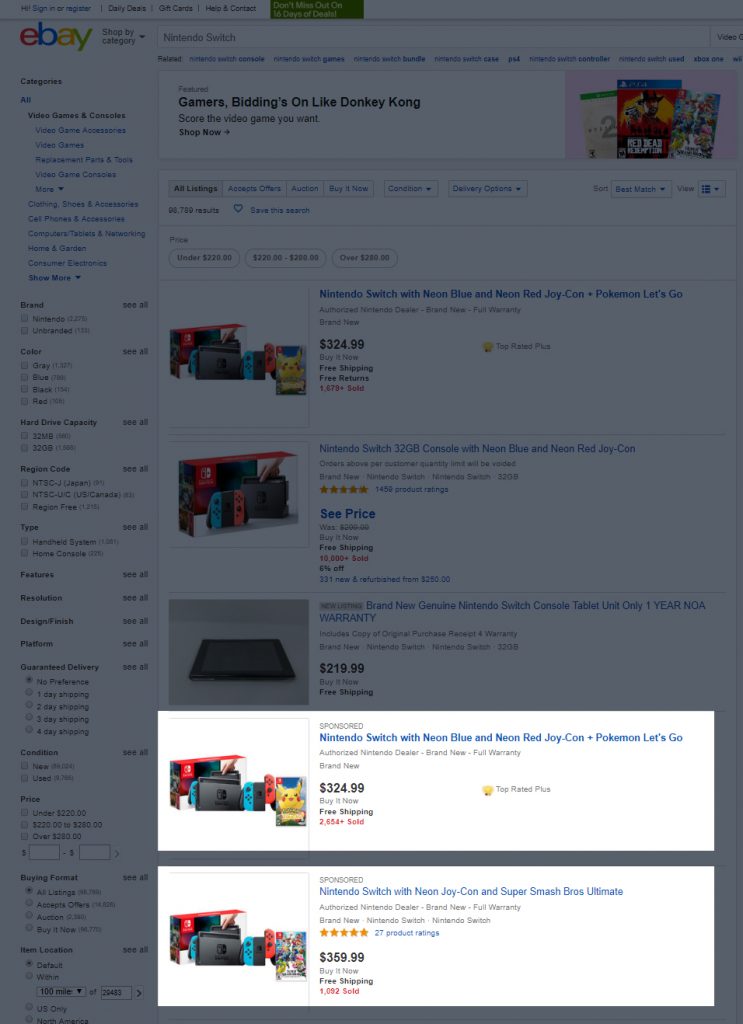The web page displayed is a dark-themed eBay listing page, primarily featuring multiple item listings. The focus of the page appears to be on cameras, with users engaged in active bidding, reminiscent of the competitive nature of "Donkey Kong." Prominently featured are two listings for a Nintendo Switch, both appearing identical in images. Despite their similarity, one is priced slightly higher than the other. The less expensive listing has a "Top Seller" badge, indicating it is from a highly reputable seller.

The page design includes a sidebar that provides helpful ideas and suggestions, though the text here is grayed out and difficult to discern. The main section of the page is filled with various listings from different sellers. At the top, the iconic eBay logo is visible, with its distinctive color scheme: a red 'e', a blue 'b', a yellow 'a', and a lime green 'y'. Adjacent to the logo, there is a search bar which users can utilize to find items across any category, enhancing the site’s navigability and user experience.